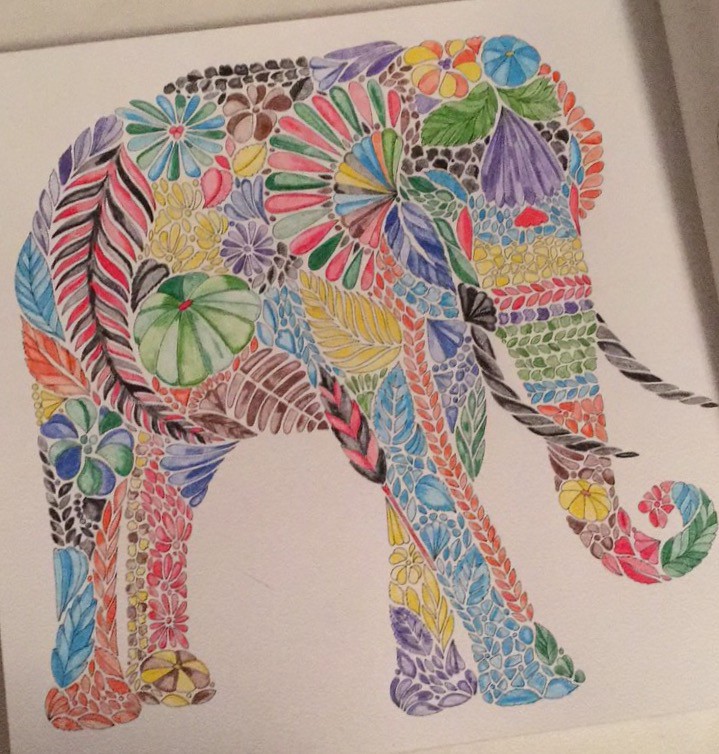The photograph showcases a drawing on a blank piece of notebook paper, perfectly framed in a square format. In the top right corner, the crease of the notebook's binding is visible, hinting at the page's origin. The opposite page of the notebook casts a dark grey shadow, creating a contrast that highlights the drawing itself. The notebook is oriented diagonally, with the top edge pointing towards the top left corner.

Central to the page is an intricately outlined adult elephant, distinguished by its long tusks. This elephant is not a simple silhouette; rather, its form is composed of a myriad of leaf and flower shapes, each representing different species. These botanical elements are vividly colored in a spectrum of hues including shades of yellow, blue, pink, purple, and green, giving the drawing a vibrant, mosaic-like appearance. The detailed textures and rich colors bring the drawing to life, offering a visually captivating experience.